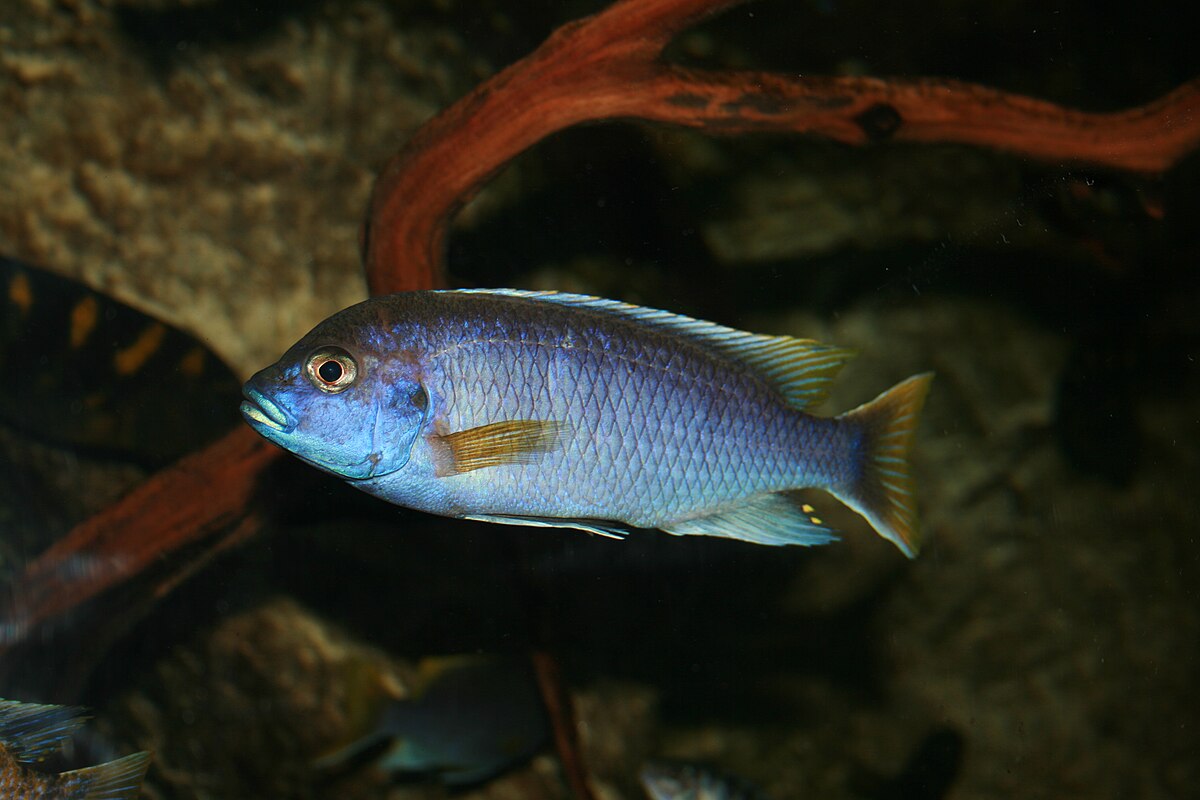In this high-quality, underwater photograph taken in what appears to be an aquarium, a stunning blue fish with iridescent, metal-flake-like scales is the focal point. Positioned in an almost perfect side profile and looking to the left, its striking black eye is encircled by a light grey ring. The fish's fins are a vibrant combination of yellow and white stripes, adding to its colorful appearance. In the background, the environment features ornamental elements like a curvy driftwood branch anchored into the water, along with brown rocks that suggest a natural underwater habitat. Some orange, irregularly shaped plants grow around, enhancing the oceanic feel. The lower left corner reveals partial fins of another similar fish, hinting at a small school. The overall scene is darkly lit, likely requiring the use of a flash, which illuminates the fish brightly against the subdued backdrop, emphasizing its detailed and glossy features.